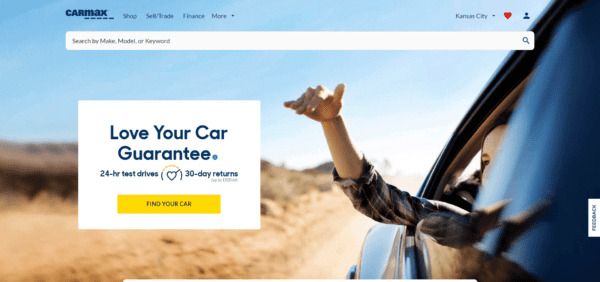Here is a detailed and cleaned-up descriptive caption for the image:

---

This web page from CarMax features a horizontal rectangular layout. At the top left corner, the CarMax logo appears in bold navy blue letters. To the right, there are navigation options labeled "Shop," "Sell/Trade," "Finance," and "More," which includes a dropdown arrow. On the far right, the page indicates the location "Kansas City" accompanied by a red heart and a person icon symbolizing a user account.

Below the navigation bar, a prominent white search bar invites users to "Search by make, model, or keyword." The background of the entire page is a photograph depicting a young girl sitting in the back seat of a moving car on a desert road. She is a white person with her arm extended out of the window, playfully catching the air with her hand. She is wearing a plaid shirt in shades of brown and cream. Her arm is slender, with delicate features visible in her forearm, wrist, and hand. The vehicle appears to be a dark-colored sedan.

Adjacent to her hand, a white box contains the text "Love Your Car Guarantee" in blue. Below this, it mentions "24-hour test drives, 30-day returns" in smaller font. A yellow box beneath this information includes the prompt "Find Your Car" in blue text.

---

This caption ensures clarity and provides a vivid description of the web page and the photograph it features.